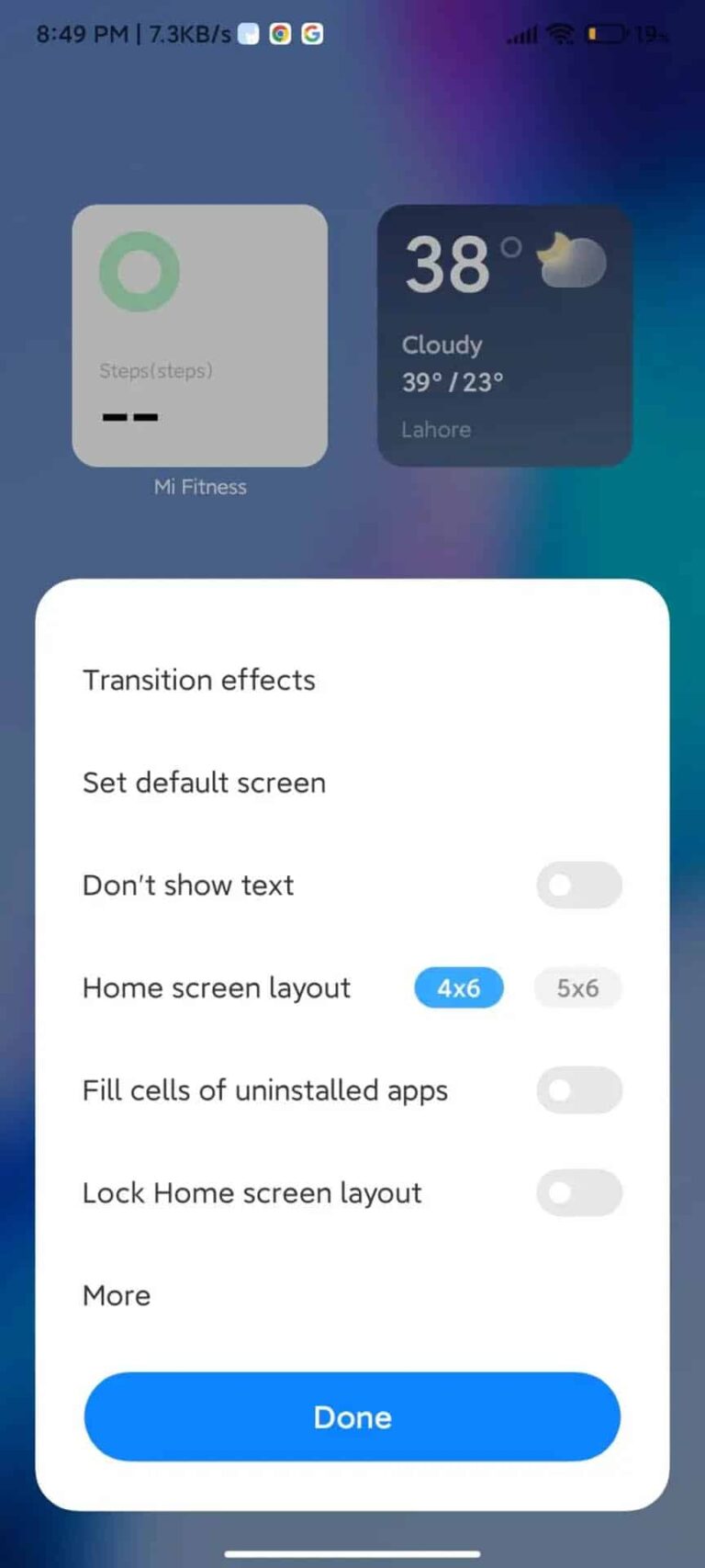A screenshot of a mobile device, taken at 8:49 p.m., displays various details. The device shows a data transfer rate of 7.3 kbps. Google Chrome is open, and the battery level is critically low at 15%. The background features a gradient of blue and purple hues.

Prominently, two widget boxes are visible. The first widget is a fitness tracker labeled "My Fitness," displaying a green circle with step count lines. The second widget is a weather box showing a nighttime forecast with a cloud and moon icon. It lists the temperature as 39°F (or perhaps a range of 23 to 33°C) for Lahore. The weather is described as cloudy.

Below these widgets is a settings box for home screen options, offering choices such as "Transition effects," "Set default screen," and "Don't show text," which is currently deselected. The layout options include a 4x6 grid (selected) and a 5x6 grid. Options to "Fill sales of uninstalled apps" and "Lock home screen layout" are both off. At the bottom, there is a "More" button and a blue "Done" button.